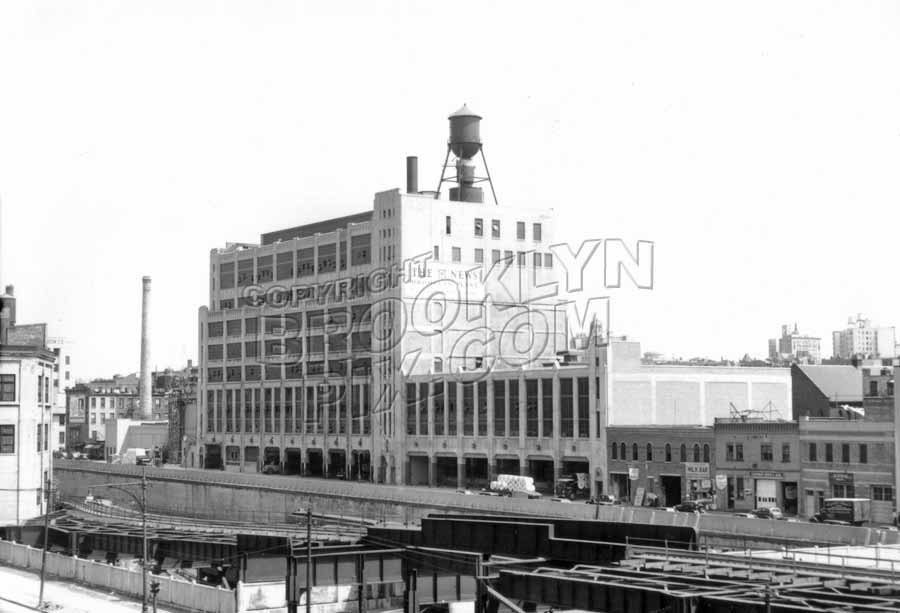This black-and-white landscape photograph depicts a city street dominated by a large, multifaceted building, likely a factory, situated under a clear sky. Central to the image is the impressive main structure, which rises to at least five stories and features an abundance of windows aligned in multiple stacks, suggesting numerous floors and significant industrial use. Atop this primary building is a distinct water tank, notable for its cone-shaped top and bottom, supported by metal framework. This tank is often mistaken for a smokestack due to its prominent placement and shape.

Adjacent to the main building, to the left, stands an actual smokestack, reinforcing the industrial atmosphere of the scene. Below the towering structures, the building facade presents multiple cutout areas resembling garage doors, eight on one level and six on another, hinting at the building's functionality and scale.

The street stretches out, lined with additional connected buildings that appear to be business premises, eventually leading to what looks like residential houses in the distant background. In the foreground, there’s an overpass, and lower to the front right, potential train tracks visible, contributing to the urban industrial setting.

The entire picture is overlaid with a curvy watermark that reads "Copyright brooklynpix.com," aligning with the vintage and historical feel of the photograph, potentially evoking a sense of nostalgia or archival documentation.